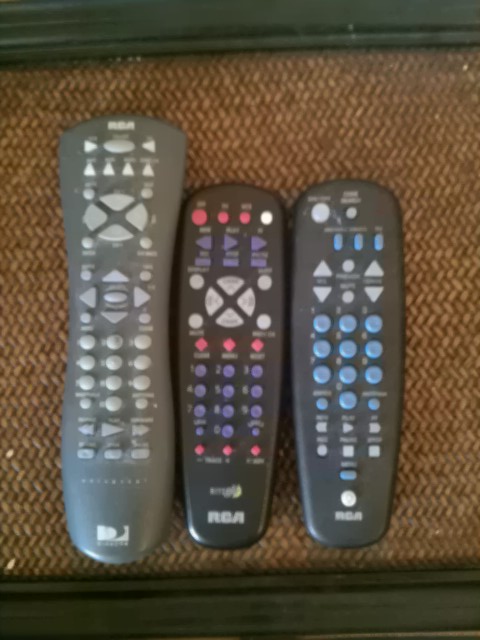Three old, vintage-style RCA remote controls are laid side-by-side on a light tan, woven fabric background, possibly a side table. On the far left is a light gray remote with matching light gray buttons, featuring the RCA logo at the top and the DirecTV logo at the bottom. The middle remote is black with multicolored buttons in shades of blue, red, and gray; it has an indistinct logo above the RCA label at its bottom. The third remote is dark gray with a mix of blue and white buttons, and it also has an RCA logo at the bottom. Despite the overall blurriness of the image, these details highlight the distinct designs and color schemes of the remote controls.